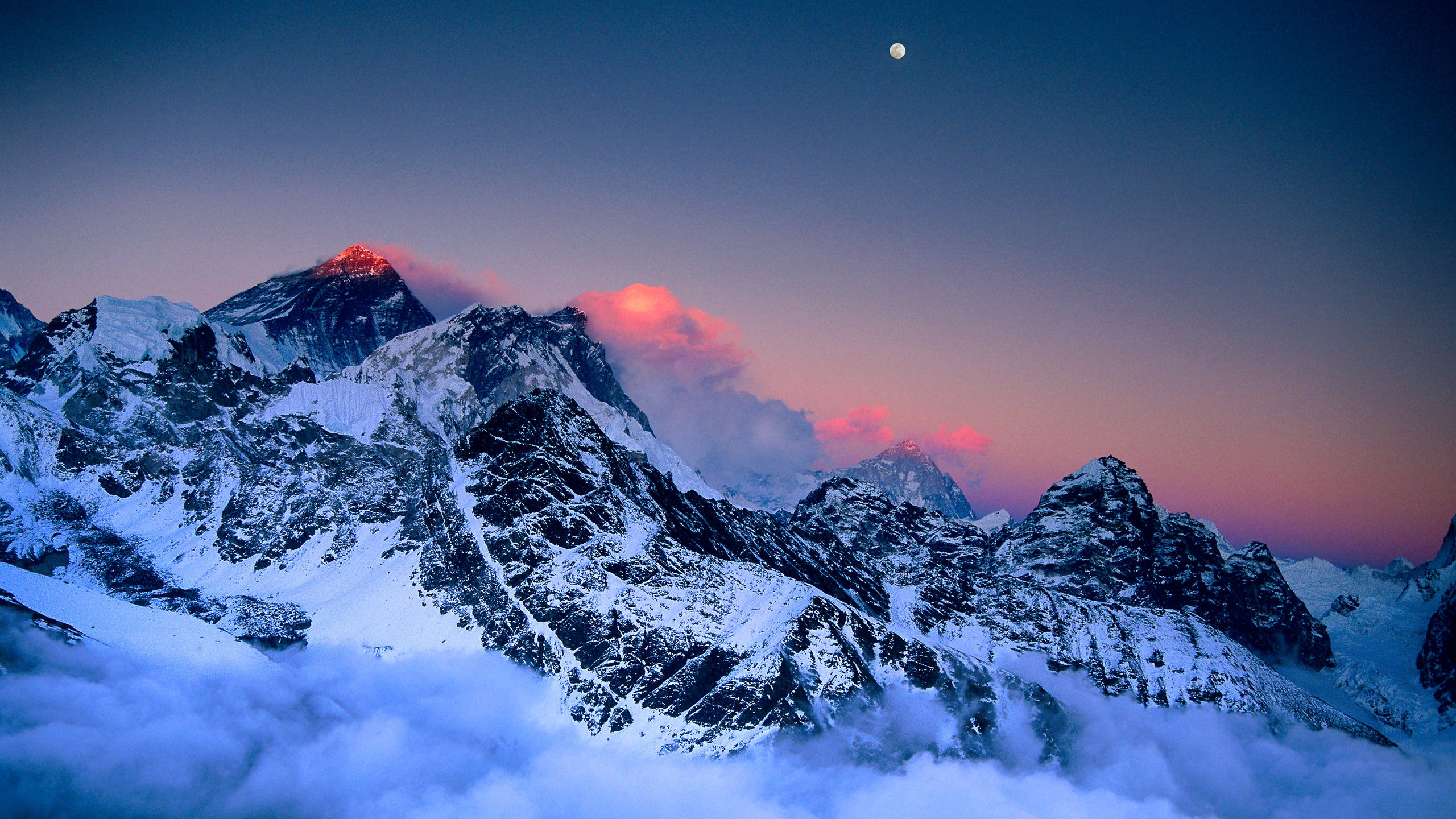In this stunning, high-altitude photograph, possibly capturing the Himalayas or Andes, we gaze upon a majestic mountain range enveloped in the ethereal beauty of dusk. The peaks, cloaked in snow, tower above a sea of clouds, which stretch across the lower half of the image. Wispy clouds meander gracefully around the summits, adding to the serene yet dramatic atmosphere. The highest peak, isolated above the dense cloud cover, is kissed by the last rays of the setting sun, reflecting a soft peachy-pink glow that paints the surrounding clouds with an enchanting ombre effect. Above this illuminated horizon, the sky transitions from a darkening blue into an almost black expanse, highlighted by the delicate presence of a full moon hanging low in the top center of the frame. The contrast of dark basaltic rock and pristine snow, textured and sporadic across the mountains, enhances the rugged grandeur of the scene, making this a breathtaking portrayal of nature's sublime beauty at twilight.